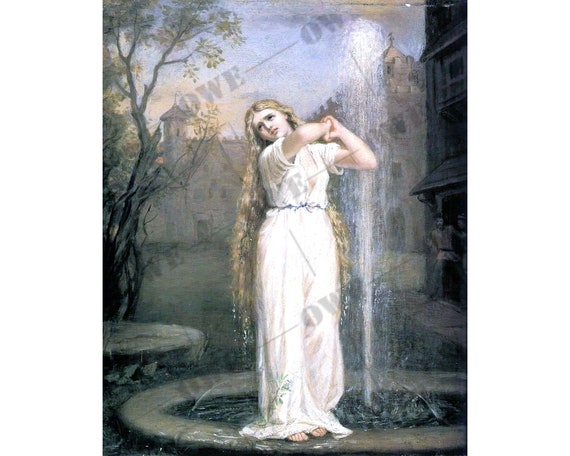The image depicts a delicate painting of a young woman from possibly the late 1700s or early 1800s, standing on the edge of a fountain. She is adorned in a long, flowing white dress that drapes past her feet, with her toes just visible. Her long, blonde, wavy hair cascades down to her knees. The woman stands with her head tilted to the right, arms raised and clasped together above her right shoulder, perhaps gesturing or reaching back. Behind her, the fountain's spout jets upward, raining water around her, and reaches about 25-30% taller than her. The background features a partly cloudy daytime sky, a tree on the left, and cityscape elements including large buildings and smaller structures. Two figures can be seen standing near a building, watching her. The soft, pale colors of the painting add to its historical ambiance.